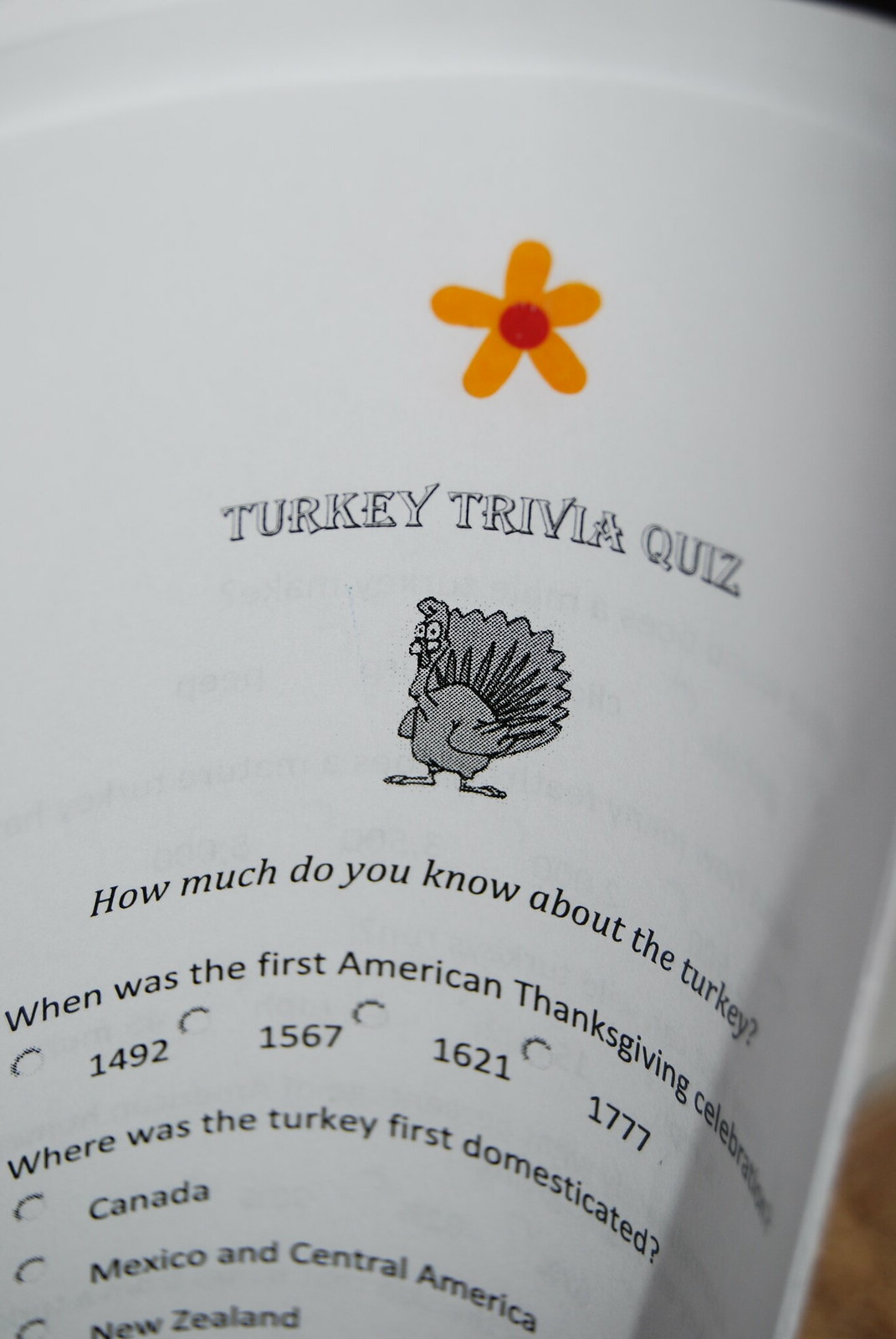The image is a photograph of a printed Turkey Trivia Quiz. At the top of the page, there is a hand-drawn orange flower with five petals and a red center, likely created with a marker. Below this, the title "Turkey Trivia Quiz" is prominently displayed. Accompanying the title is a black and white clip art image of a cute turkey with a charming face. The quiz begins with the question, "How much do you know about turkey?" followed by the first question: "When was the first American Thanksgiving celebration?" The options provided are 1492, 1567, 1621, or 1777, each with a checkbox next to it. The subsequent question is "Where was the turkey first domesticated?" with options including Canada, Mexico and Central America, and New Zealand. The document appears to be slightly curled, suggesting it is either being held in someone's hand or possibly printed on a curved surface, like the side of a cup. A section of the right-hand side of the image reveals a brown patch, possibly indicating a table or wooden surface.